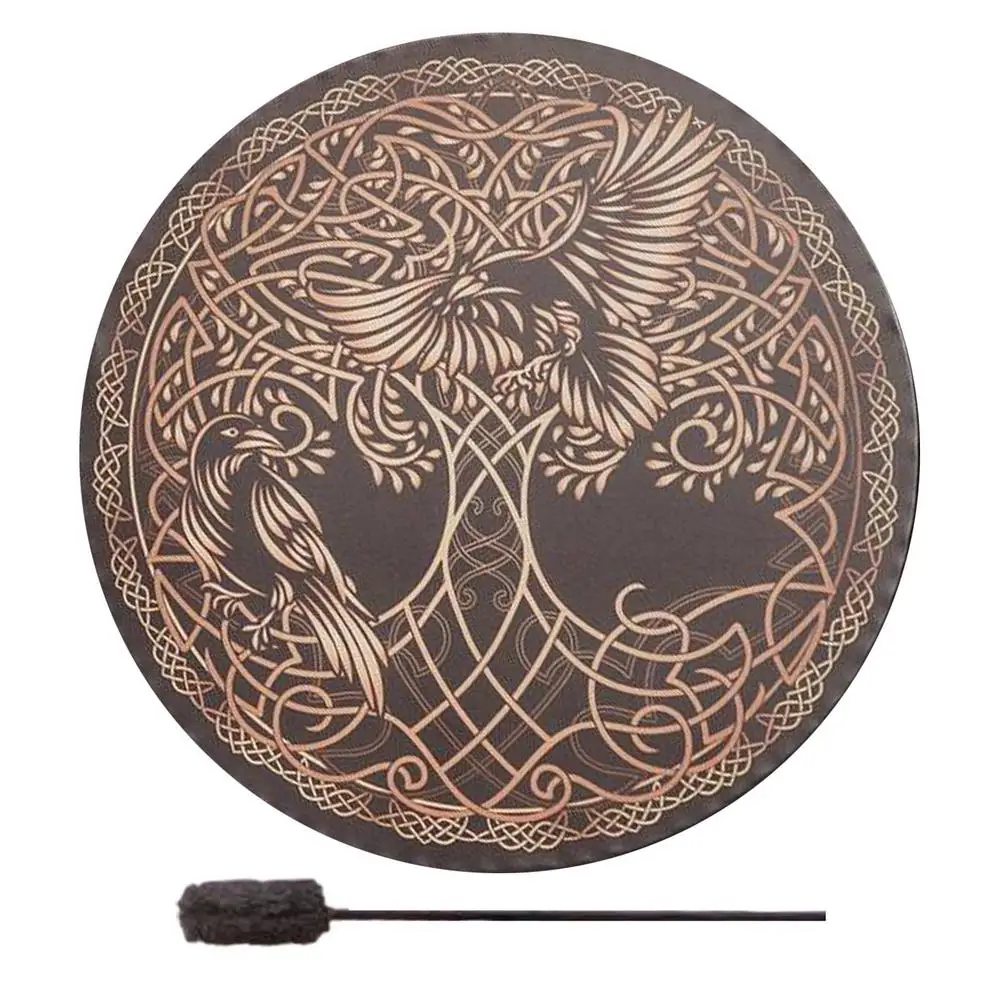This image displays a large, round plaque, possibly a drum or shield, made from a dark-toned material—either wood or steel-looking surface with a chocolate brown background. The plaque is intricately adorned with a Celtic-inspired design, featuring the Tree of Life at its center. Flanking the tree are two black birds; one bird is in flight while the other perches, each with distinctive white wings and tail feathers. The central motif is encircled by elaborate knotwork and scroll-like patterns in varying shades of brown, gray, and off-white. Beneath the plaque lies a black stick with a fuzzy, cloth-like tip, which could serve as a drumstick or potentially as a torch.